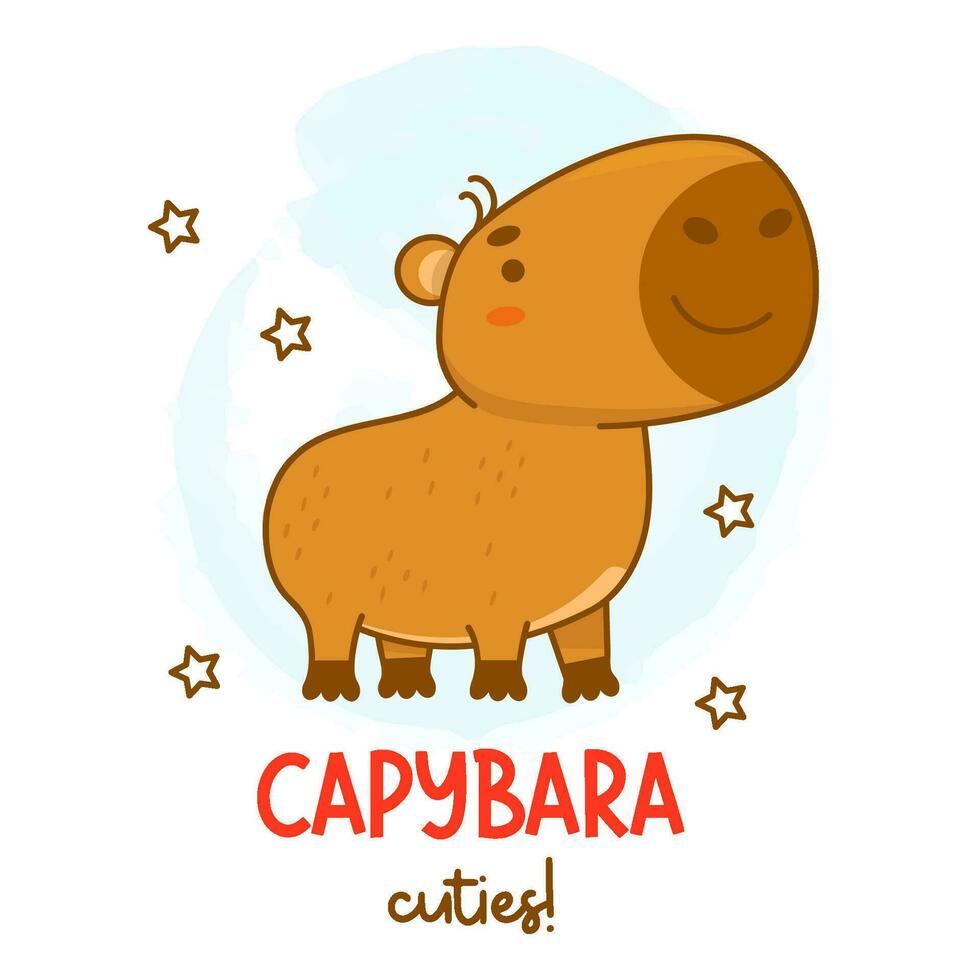The image is an illustration of a capybara, designed with a whimsical, children's book style. In the center, a large, rodent-like capybara is positioned with its head turned slightly to the right. The capybara has a light brown body and head, with darker brown feet and snout. It features two small nostrils, a curved smile, a black eye with a dark brown eyebrow, two curved lines that suggest hair, and a round tan-colored ear. The capybara stands against a baby blue and white background, placed inside a small blue circle. Surrounding the capybara are five small brown circles, resembling stars, with three to the left and two to the right. At the bottom of the image, large red text reads "capybara," and below it, smaller cursive brown text reads "cuties." The charming look of the capybara, along with its simple, child-friendly design, creates an overall cute and inviting visual.